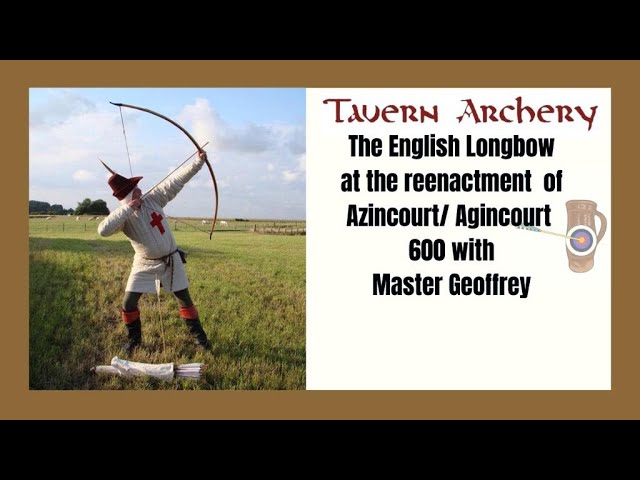This advertisement for Tavern Archery showcases a reenactment of the Battle of Agincourt on its 600th anniversary, featuring Master Geoffrey demonstrating the English Longbow. The image appears to be a screenshot of a video or a PowerPoint slide, framed by black bars at the top and bottom. The layout includes a tan square background with a photograph on the left and text on a white box on the right.

In the photograph, set against a lush green field on a sunny day, a man dressed as an English archer stands poised, drawing his bow. He wears a white tunic with a prominent red cross on the chest, symbolizing England, and a cavalier-style hat with a feather, evoking a Robin Hood-like appearance. The man's outfit includes green stockings with boots accented in red around the cuffs, and a quiver of arrows rests by his feet.

The accompanying text, styled in an old English font, reads "Tavern Archery" in red, followed by "The English Longbow at the Reenactment of Agincourt 600 with Master Geoffrey" in black. An old-school graphic of a target is also displayed, reinforcing the archery theme.